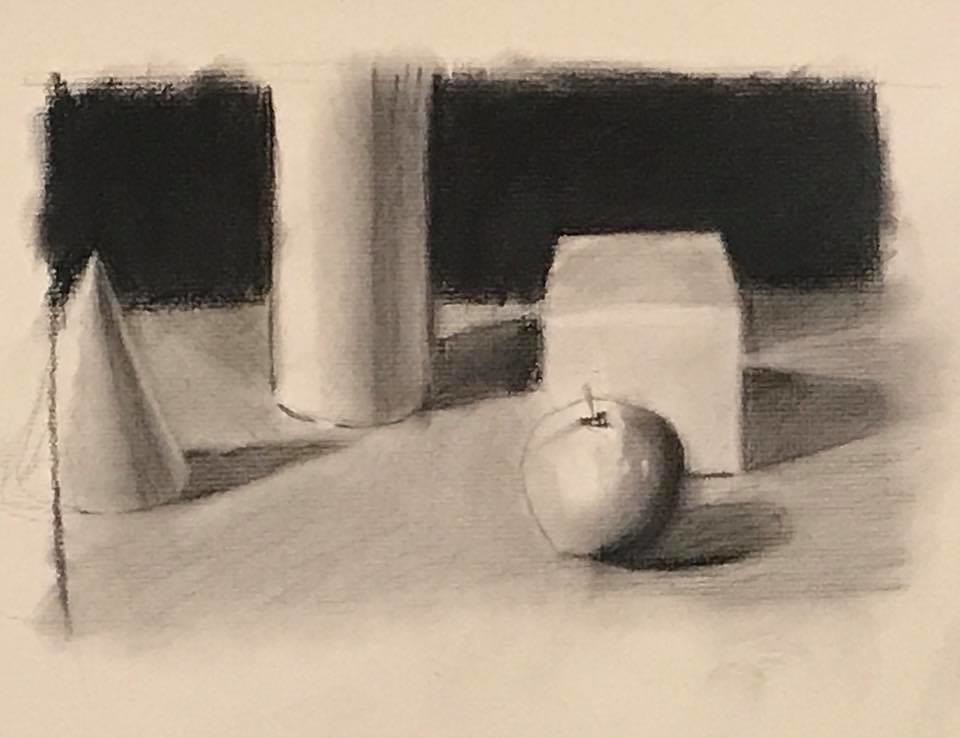This image appears to be a meticulously detailed charcoal sketch on very pale, whitish-gray paper. The composition includes several objects arranged on what seems to be a flat surface, either a table or floor. Each item is accompanied by a distinct shadow, adding depth and realism to the scene. Dominating the background is a stark black charcoal rectangle, which provides a dramatic contrast to the lighter elements in the foreground.

In front, there is a realistically drawn apple, complete with a stem, capturing the essence of its natural form. Slightly behind the apple is a white rectangular box, its sharp edges and flat surfaces rendered with precise strokes. Adjacent to the box stands a tall, cylindrical object, possibly a vase, exhibiting smooth lines that accentuate its elegant, slender shape. To the left of the vase, a short, conical form is depicted with careful attention to its geometric simplicity. Together, these elements create a study in contrasts and textures, showcasing the artist's skill in manipulating shadows and light.